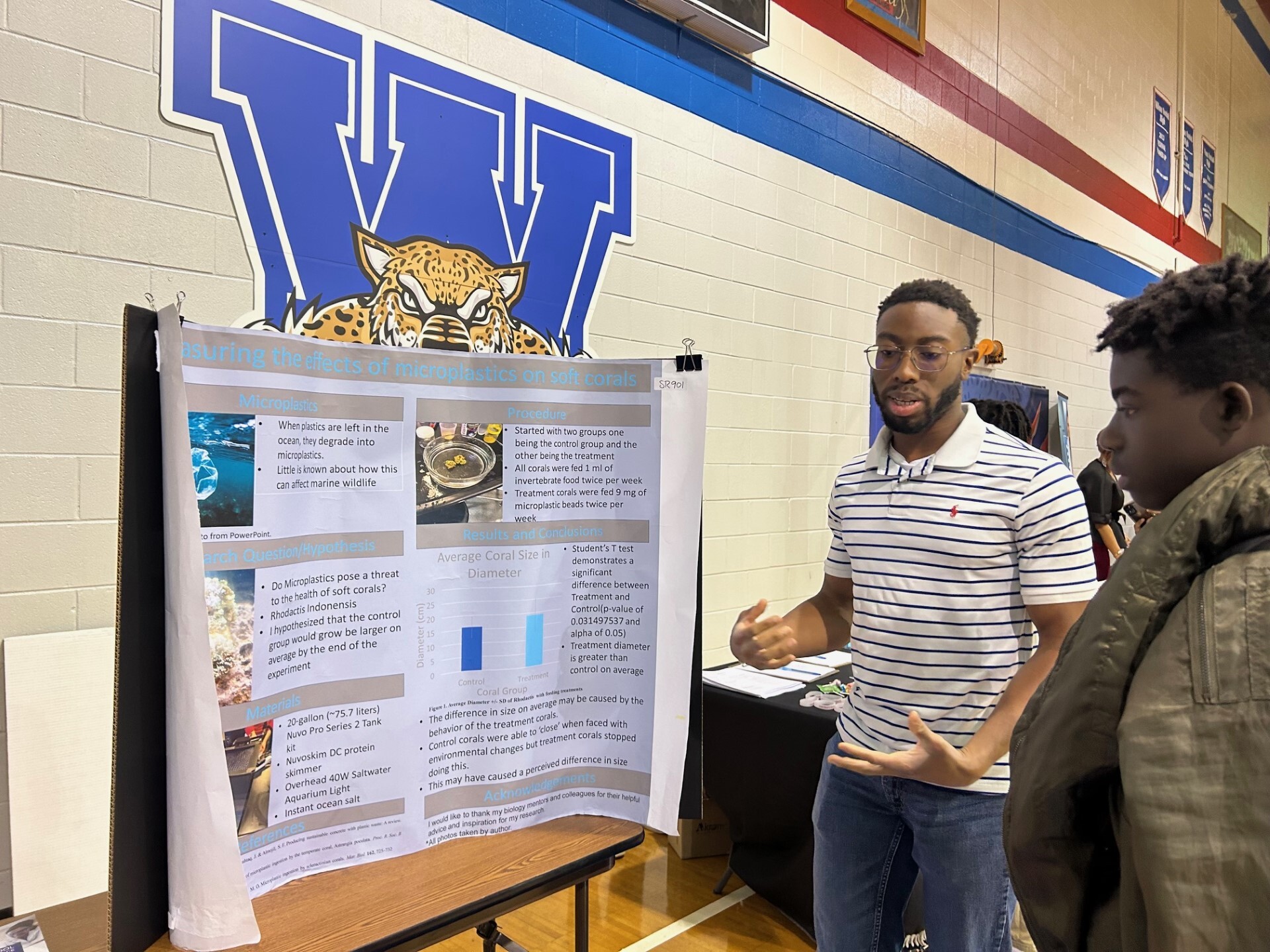The image captures a detailed scene at a high school science fair held in a gymnasium with cream-colored walls adorned with red and blue horizontal stripes. The school's partial mascot, a tiger, and a large "W" can be faintly seen in the background. The focal point is a student of African descent on the right side of the image, identifiable by his short hair, glasses, and thin beard. He is dressed in a white polo shirt with thin horizontal blue stripes, featuring a distinct red polo logo on the right chest, paired with light blue jeans. This student seems to be explaining his project on "Measuring the Effects of Microplastics on Soft Corals" to another student, who is also of African descent and wearing a green puffy jacket. The science fair is bustling with activity as other students wander around, examining different projects displayed on tables throughout the gymnasium.